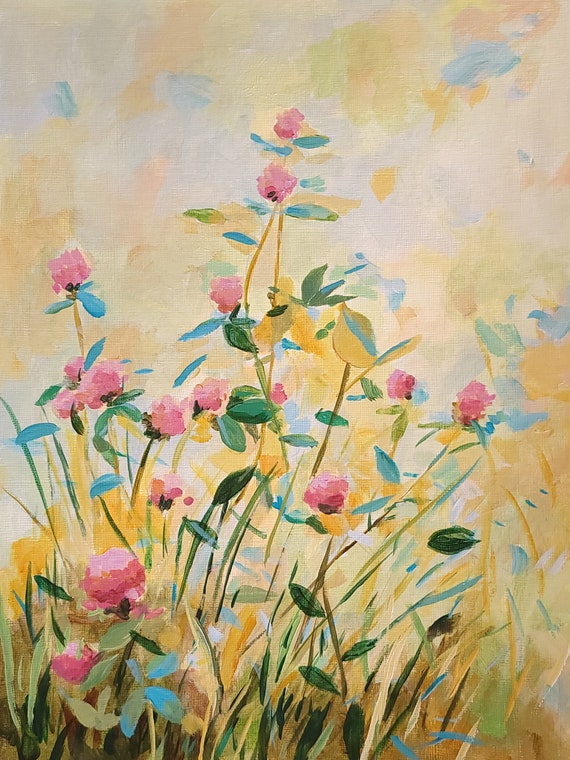This rectangular painting, approximately six inches high and three to four inches wide, is a colorful representation of a garden, captured on a textured canvas that exhibits noticeable left-to-right threading marks. Utilizing what appears to be acrylic paint, the artist has created a detailed and vibrant composition. 

The foreground features a slightly chaotic yet enchanting array of tall vertical stalks, blades of grass, and stems adorned with pink and yellow flowering buds. These plants are depicted in a range of hues including dark green, light green, off-tan, and darker tan, while some of the leaves exhibit a striking light blue color. The bottom is filled with a tangle of tall, curved grass blades and plant stems, evoking a sense of wild growth.

The background is warmly colored, dominated by gold and cream tones with hints of pale blue suggesting a sky dotted with cream and white puffy clouds. This warm palette enhances the romantic and somewhat abstract feel of the piece, which lacks any visible signature. The overall style is reminiscent of garden art or romantic abstract art, characterized by its slightly chaotic yet carefully detailed, colorful depiction of a blooming garden.